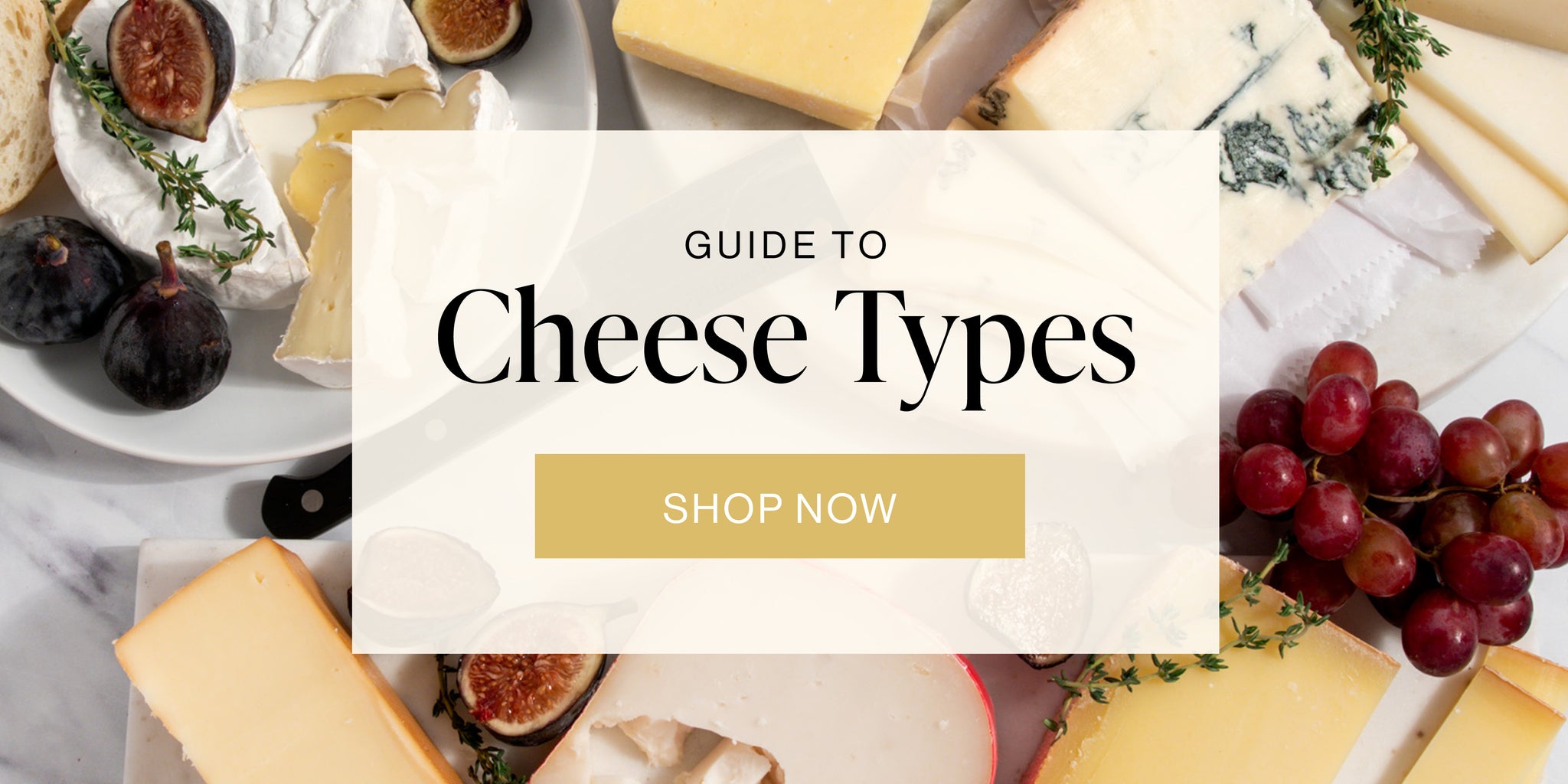This vibrant advertisement, potentially a promotional insert or the front of a magazine, prominently features a creamy white rectangle in the center. The rectangle contains bold text that reads "Guide to Cheese Types" — with 'Guide to' in smaller lettering above 'Cheese Types' in larger font. Beneath this heading is a gold-colored button that says "Shop Now" in white font. The button appears clickable and adds a call-to-action element to the image. Behind this text overlay, a beautifully arranged cheese board catches the eye, set against a white surface with subtle cloth accents. The display includes various types of light yellow cheeses, possibly including brie and blue cheese, along with purple grapes, figs, and slices of bread, all artfully placed on a white plate. There might also be a hint of a cheese knife peeking out, emphasizing the ready-to-enjoy nature of this delectable spread.